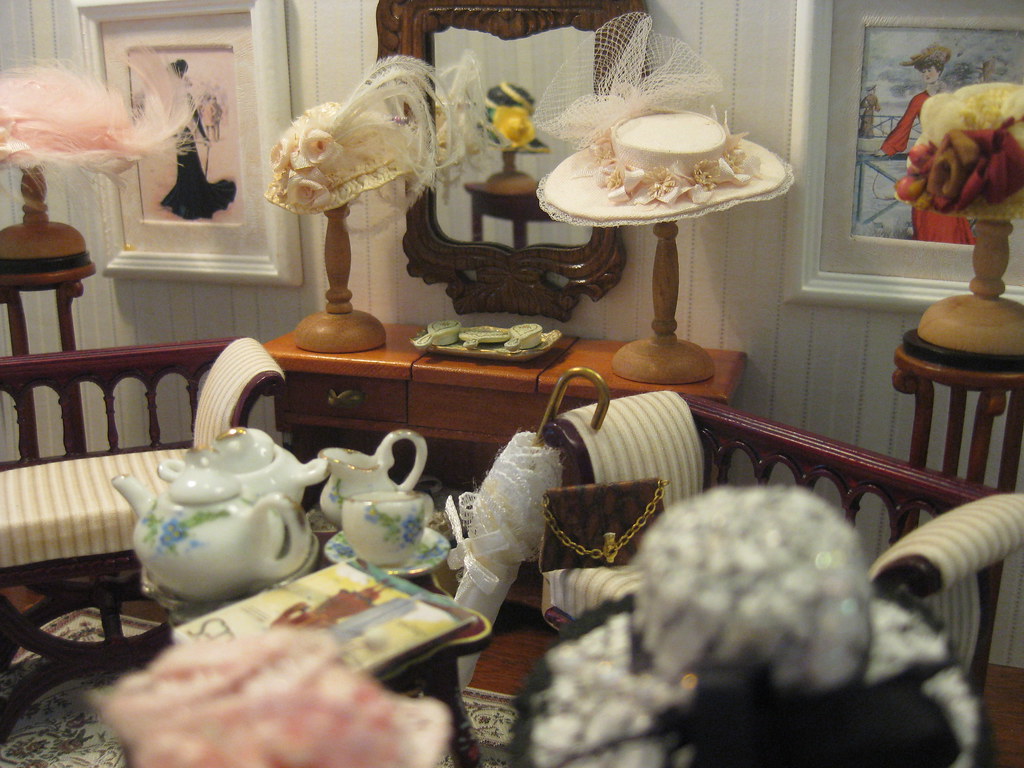This image captures the inside view of a very cluttered room that might belong to a dollhouse, giving off a plasticky feel. The back wall is adorned with white-painted wooden slats arranged as vertical stripes, creating a contrasting backdrop for the décor. Central to the back wall is a mirror with a brown border, flanked on either side by white-framed pictures of women in old-fashioned, ornate dresses—one in black on the left and the other in red on the right.

Below the mirror sits a brown desk that acts as the room's central furniture piece. This desk features two small brown cylindrical vases at its ends, each holding a hat: a yellow and white one on the left and a flat-brimmed pink one on the right. In front of the paintings, there are two more hat stands, with a pink feathered hat on the left and a yellow hat adorned with red flowers on the right.

To the left of the desk, partially cut off by the edge of the image, stands a red wooden chair featuring a white cushion with brown stripes. The foreground showcases a wooden table set for tea, adorned with a white and green-blue floral designed teapot, creamer, sugar bowl, and teacups. To the right of this tea set lies a white umbrella with a gold handle. Beside the umbrella, there is an identical chair to the one described earlier, topped with a brown purse featuring a gold chain.

Right in front of the camera, slightly out of focus, is a black and white hat embellished with a large black bow. Scattered nearby on the table are a stack of magazines, featuring two women on the cover, although the title remains unreadable. The room is brimming with intricate details and appears meticulously arranged, despite its busy nature.